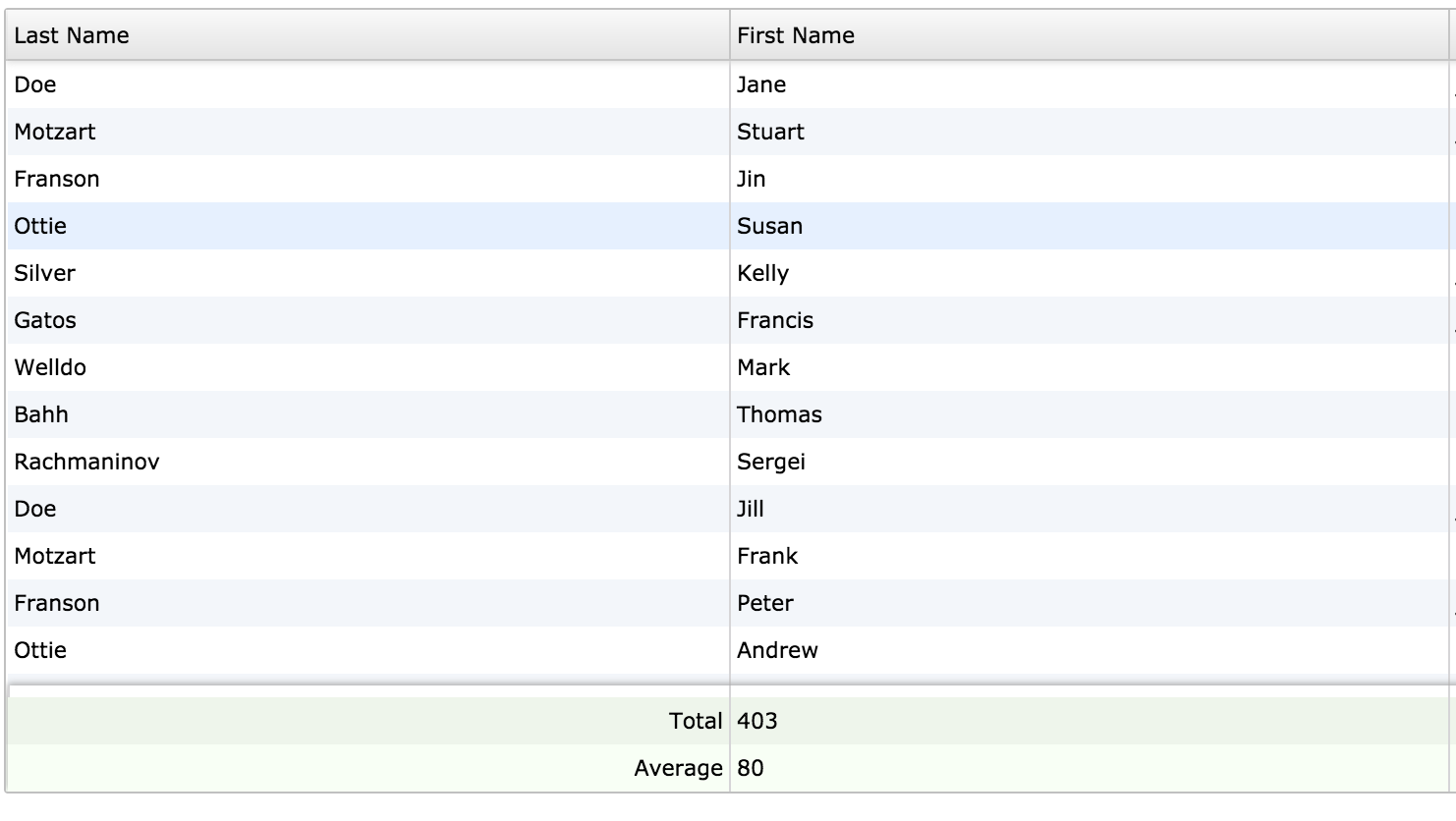In the upper left corner of the image, there is a long rectangular section labeled "Last Name" with a gray background. To its right, there is another gray-background rectangle labeled "First Name." Underneath "Last Name," there is a vertical list of names: Doe, Mozart, Franzen, Otti, Silver, Gatos, Welledoe, B-A-H-H, R-A-C-H-M-A-N-I-N-O-V, Doe, Mozart, Franzen, and Otti. Parallel to this, under "First Name," the list includes: Jane, Stewart, Jen, J-I-N, with a notable entry highlighted within a blue-background rectangle named Susan. Continuing down the list are the names: Kelly, Francis, Mark, Thomas, Sergei, Jill, Frank, Peter, and Andrew. At the bottom of the image, there is a long, light-gray rectangular section featuring the word "Total" with the number 403 beside it. Additionally, below this, the word "Average" is accompanied by the number 80.